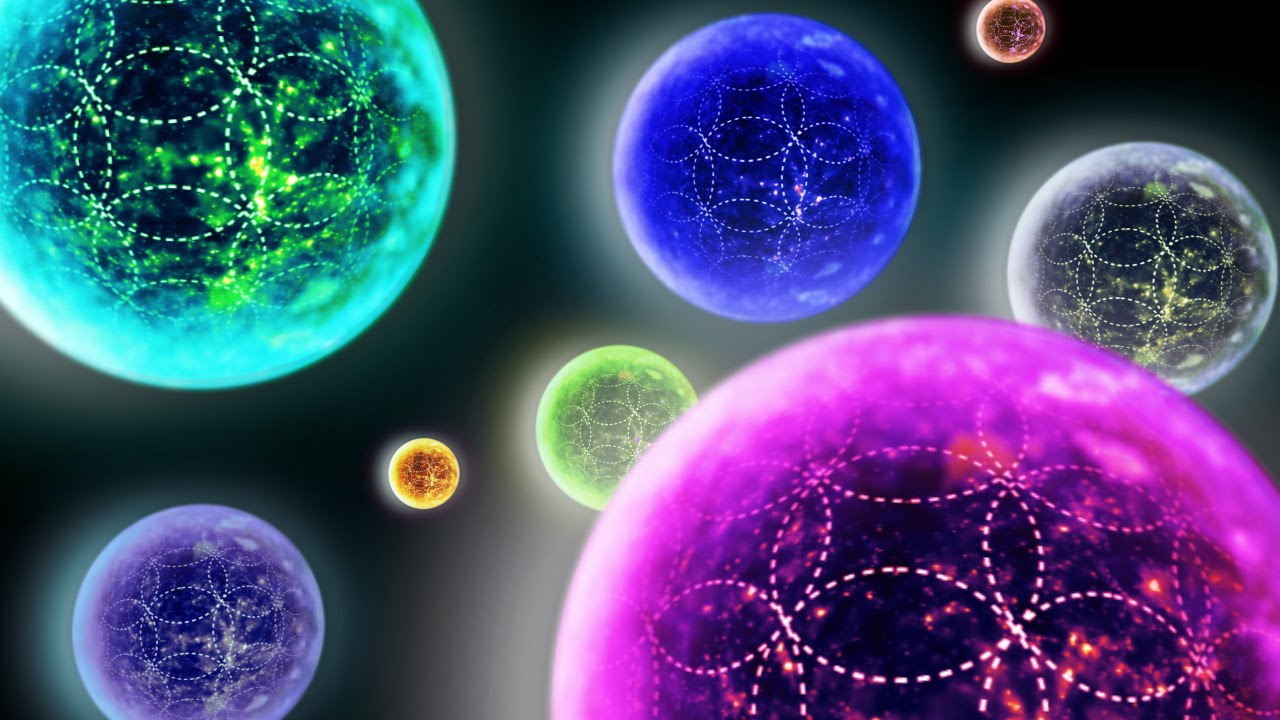This rectangular, computer-generated image, oriented in a landscape layout, features a surrealistic portrayal reminiscent of the solar system, but instead showcases a variety of colorful, semi-transparent spheres suspended in a black, night-sky-like background. These spheres vary in size, with the largest positioned in the bottom-right corner, displaying a vibrant pink-purple hue and only half visible. Each sphere emits a distinct glow, surrounded by a ring of light that enhances their ethereal appearance.

The spheres exhibit intricate, swirled patterns formed by broken lines that match their respective colors. Among the array, notable ones include a green sphere in the top-left corner, partially cut off, showcasing an aqua outer edge with a floral-like design in light green; a dark blue sphere near it with a similar looping pattern; and a smaller golden-yellow sphere towards the upper right. A pinkish sphere tending towards red can be seen in the lower right, emitting a noticeable glow. Behind it lies a smaller green sphere, and slightly above, two diminutive spheres, one with a golden sheen and the other with an orange tint, complete the composition.

Every sphere's internal pattern consists of swirling dotted circles, creating intricate, overlaid designs. The entire scene is bathed in a surrealistic ambiance, with each orb glowing as though possessing its own miniature cosmos within.